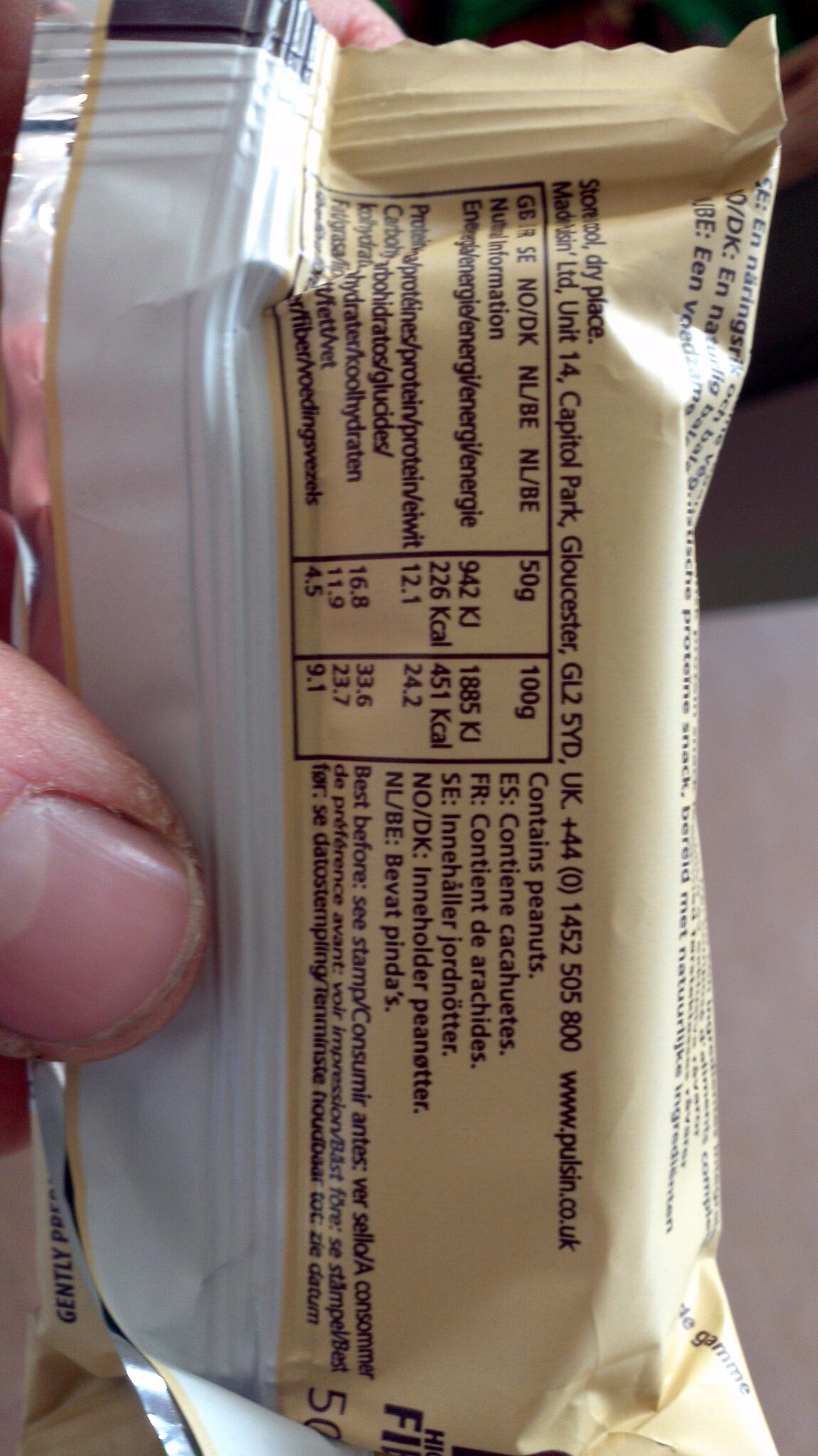This image features a close-up of a person's thumb holding the back of a Pulsin protein bar package vertically. The tan and white wrapper, with beige and slight yellow hues, exhibits nutritional information and multiple translations—including Spanish, French, and possibly Swedish—indicating it contains peanuts. The thumb, with an uncut nail, is prominently displayed in the foreground, while the bar is sealed at both ends, creating a ruffled edge. The text includes values in grams, kilojoules, and kilocalories, common in British English labeling, and mentions the bar’s British origin with a website link, www.pulsin.co.uk. The background transitions from a lighter pinkish lower half to a darker upper half, adding to the contextual detail of the scene.